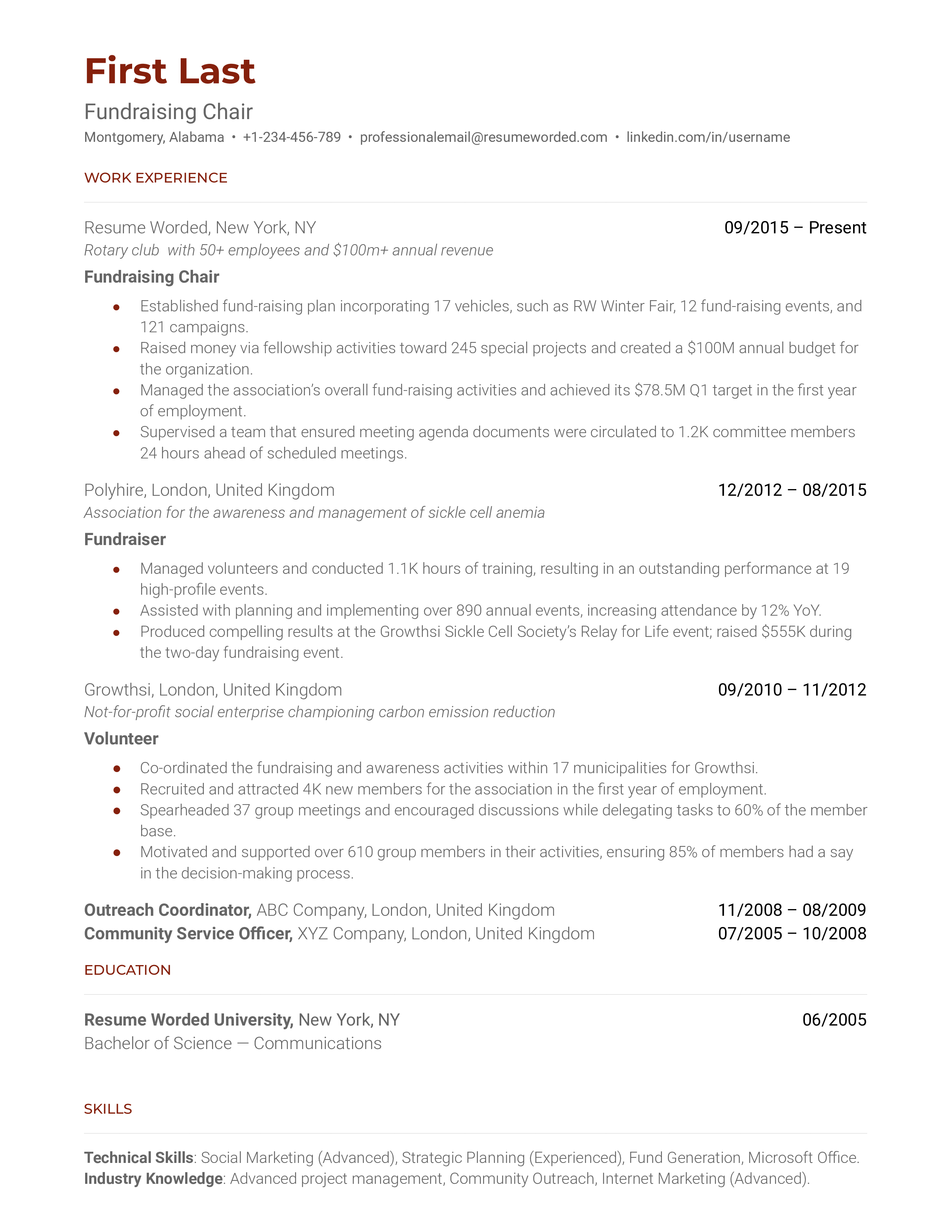The image is a digitally created resume set on a white backdrop, featuring a combination of brown, dark maroon, light black, and dark gray text. At the top left, the largest text reads "First Last," followed by the position title "Fundraising Chair" based in Montgomery, Alabama, along with a phone number, a professional email at resumeworded.com, and a LinkedIn URL. The resume details an extensive work history, including:

- **Fundraising Chair at Resume Worded, New York, NY (September 2015 - Present)**
- **Volunteer at Polyam, London, United Kingdom (December 2012 - August 2015)**
- **Outreach Coordinator (September 2010 - November 2012)**
- **Community Service Officer (November 2008 - August 2009)**

Additionally, the resume notes an educational achievement of receiving an award from a university in June 2005, and concludes with a section listing various skills. This resume could potentially be an example template for a resume company, given the placeholding nature of the name "First Last."